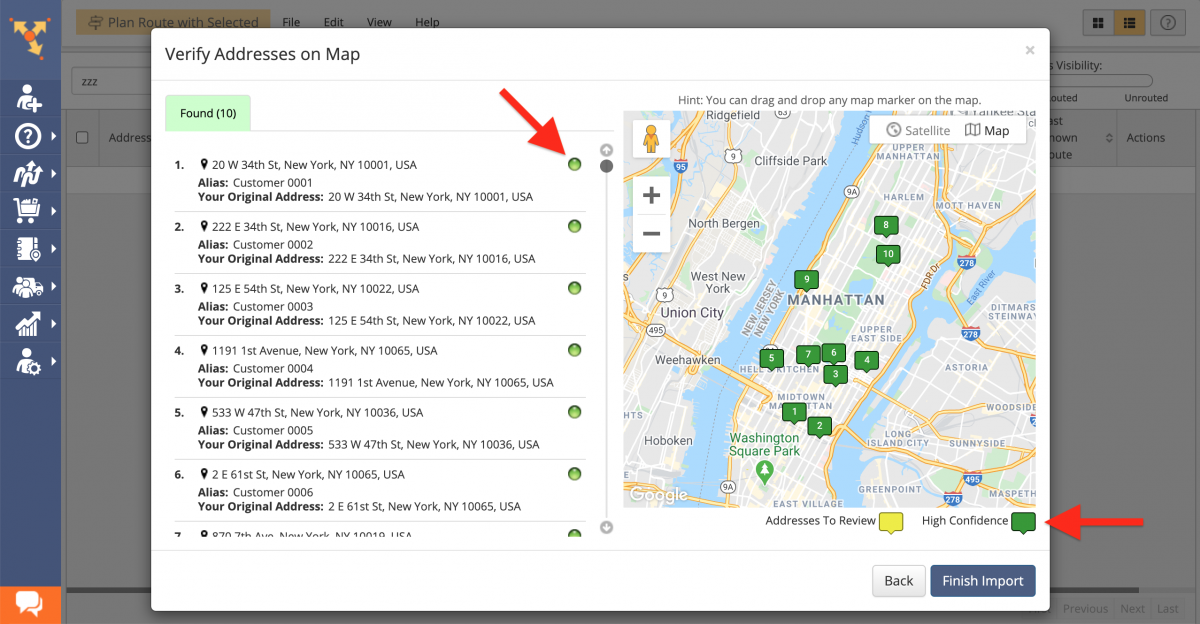The screen displays a map of Manhattan on the right side, presumably sourced from Google Maps or a similar application. On this map, approximately 10 numbered green icons are scattered, indicating specific locations solely within the Manhattan area, spanning vertically from north to south. Surrounding areas of New York are visible, but the icons are focused on Manhattan to Long Island. 

On the left side of the screen, there is a list of six visible addresses. These addresses are:

1. 20 West 34th Street, New York, NY 10001, USA
2. 222 East 34th Street, New York, NY 10016
3. 125 East 54th Street, New York, NY 10022
4. 1191 First Avenue, New York, NY 10065
5. 533 West 47th Street, New York, NY 10036
6. 2 East 61st Street, New York, NY 10065

Each of these addresses is accompanied by an alias listed right below it, correlating to their respective numbering. For instance, the first address shows "alias customer 0001," the second "alias customer 0002," and so forth.

At the bottom right corner of the screen, there are two prominent buttons labeled "Back" and "Finish Import," providing navigation options for the user.